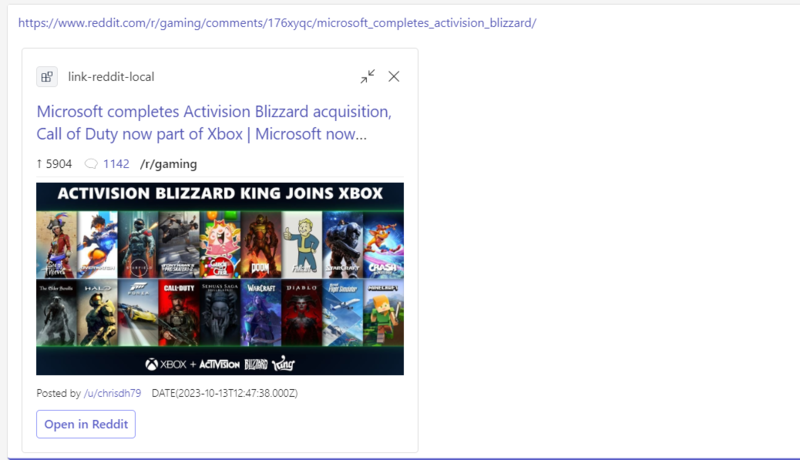Screenshot of a Web Redirect Page for a Reddit Post:

The top bar displays the URL: HTTPS://www.reddit.com/r/gaming/comments/176XYQC/Microsoft_completes_Activision_Blizzard.

The header includes navigation elements such as two arrows pointing at each other and an 'X' for closing.

The Reddit post headline reads: "Microsoft completes Activision Blizzard acquisition. Call of Duty now a part of Xbox."

A subline beneath the headline states: "Microsoft now..."

Engagement metrics show with upvoting and downvoting counts: 
- Upvotes: 5,904 
- Downvotes: 1,042

The subreddit label is "r/gaming," and there is a statement: "Activision Blizzard King joins Xbox." This is accompanied by a collage image displaying various game covers.

At the bottom of the image, there is text: "Xbox + Activision Blizzard King."

Further details include the post metadata: 
- Posted by u/ChrisDH79 
- Date: 2023-10-13T12:47:38.00Z

A button is visible for redirecting: "Open Reddit."